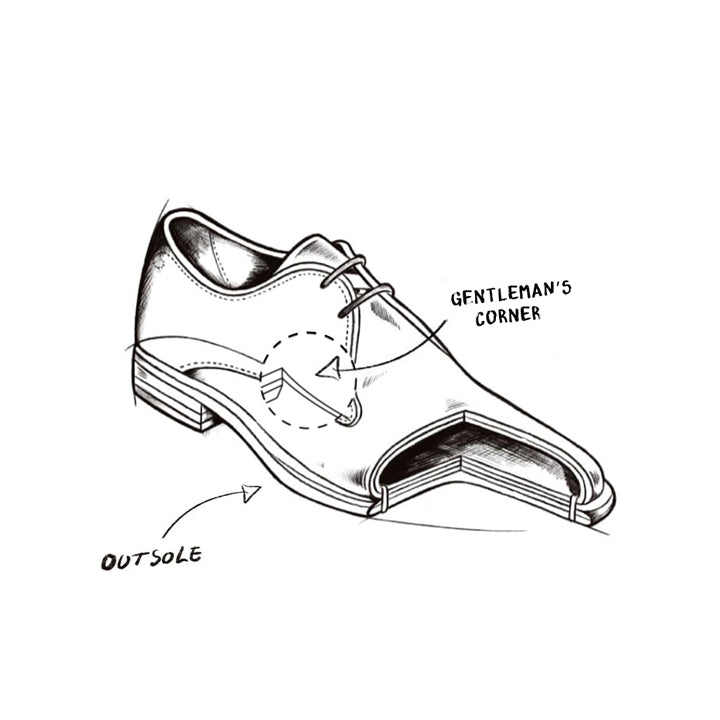This is an intricate black-on-white illustration of a classic leather shoe, executed in black pen ink. The drawing meticulously details both the shoe's exterior and interior features, showcasing its multi-layered construction. The illustration includes a cutaway section at the toe, revealing the layers of leather that make up the shoe's upper and sole. Noteworthy elements are labeled in small black text: the "gentleman's corner" in the upper right, and the "outsole" in the lower left. The shoe, which resembles a traditional Oxford loafer from the 1930s or 1940s, features a modest half-inch heel, two holes for shoelaces, and thin, vintage-style laces. The cutaway reveals at least three layers in the shoe's sole and additional interior details, such as stitching and construction. The shoe is rendered with a careful attention to craftsmanship, offering a comprehensive view of its design and construction.